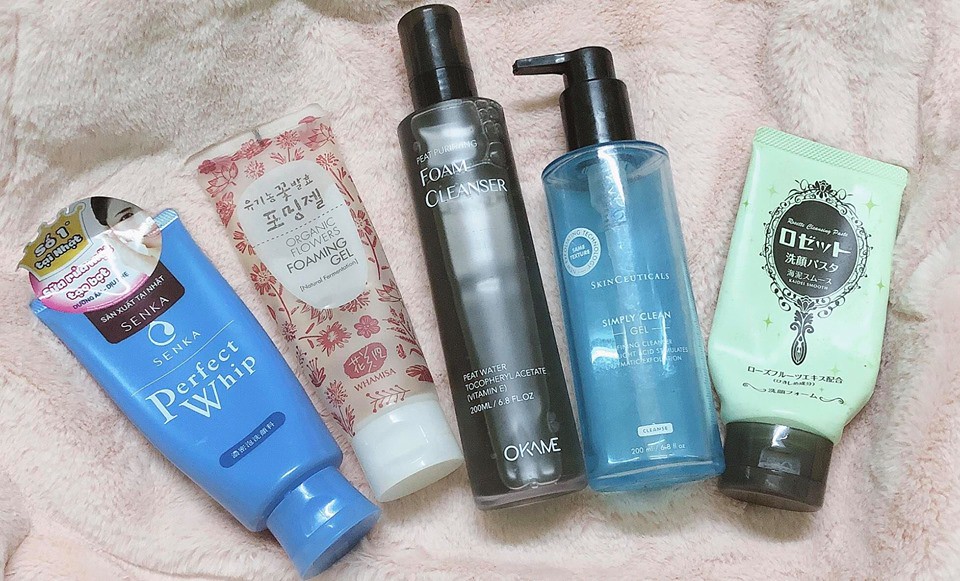This photograph captures an assortment of bathroom toiletries meticulously arranged on a plush, fluffy towel with a pinkish hue, taken from an overhead, landscape perspective. 

To the left of the frame, a blue squeeze bottle prominently displays the words "Perfect Whip" with "SENKA" underneath, and is adorned with either Japanese, Chinese, or Korean characters. 

Adjacent to it is a pink squeeze bottle capped with white, labeled "Organic Flowers Foaming Gel," alongside a multitude of Asian characters and the brand name "WHAMISA" prominently at the bottom. 

Central to the arrangement sits a dark gray bottle with a black cap, marked with "peat purifying foam cleanser." This bottle indicates the inclusion of peat water and tocopheryl acetate Vitamin E, specifying its volume as 200 milliliters or 6.8 fluid ounces.

Next, a light blue bottle featuring a convenient pump mechanism is labeled "Simply Gel."

Finally, at the far right, a very light green bottle covered in unreadable characters completes the collection, adding to the international and varied aesthetic of the scene.